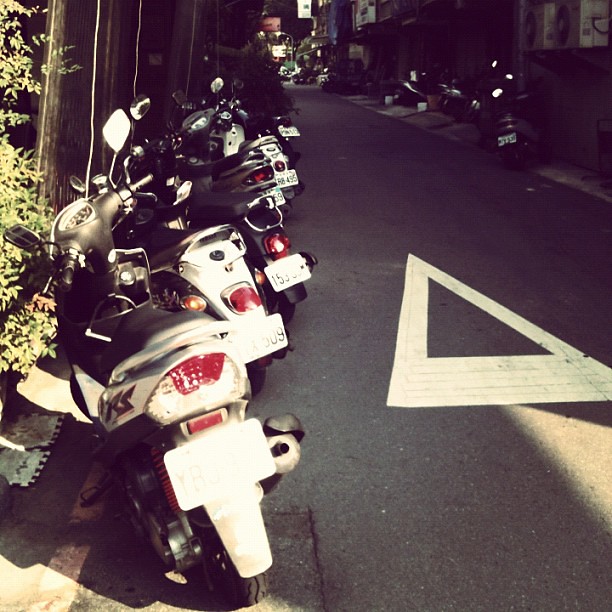This nighttime color photograph, taken with flash, captures a row of five motorcycles or scooters parked diagonally along a dark city street. The street, covered in blacktop, features a prominent large white triangle painted on it, pointing towards the top of the image. The muted and desaturated tones hint that a filter might have been applied, enhancing the high contrast between light and shadows. The motorcycles, mostly white with black seats and handlebars, have visible red taillights and are positioned predominantly on the left side of the road, with a few barely discernible on the right side due to the poor lighting. The image also shows some green foliage on the left, likely illuminated in the flash, and a drainage cement feature. In the background, air conditioning units are mounted on buildings lining the narrow street, which leads into the distance, where further shadows and structures can be faintly seen. Overall, the photograph emphasizes the desaturated ambiance and the alignment of the bikes along the street.